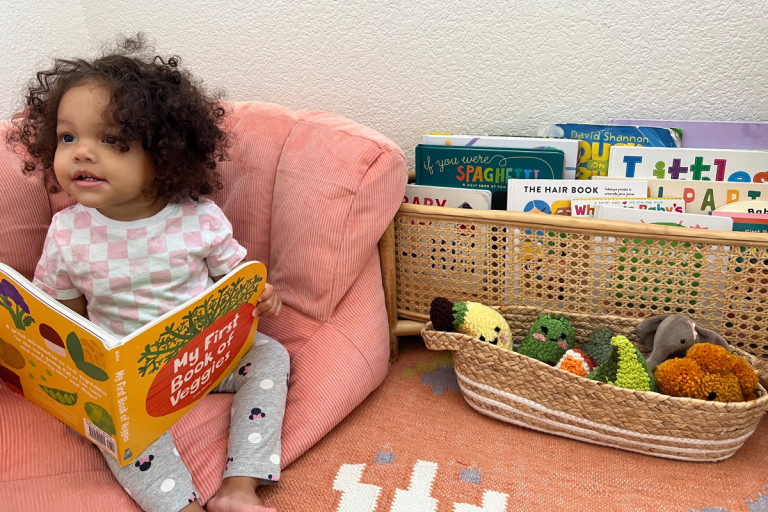This full-color, horizontally rectangular image captures a heartwarming indoor scene, likely illuminated by artificial light during the day. It features a toddler-aged Black girl with afro-like hair, sitting comfortably on a cozy, pink corduroy beanbag chair. She is dressed in a checkered pink and white top and gray pants adorned with a subtle Disney character. 

Holding an open book titled "My First Book of Veggies," which sports a yellow cover with a beet illustration, the little girl is intrigued by something off-camera rather than the book. Surrounding her, the environment is filled with child-friendly elements—an orange mat or blanket lies next to her chair, accompanied by a woven basket containing plush, hand-knit toys and another basket brimming with various little books. Notable among these books is one titled "If You Were Spaghetti." 

The backdrop is a white stucco wall with a textured finish, enhancing the coziness of the scene. The image is beautifully rich in colors, featuring light tan, off-white, light pink, gray, yellow, red, orange, light green, light blue, and light purple, creating a vibrant yet serene atmosphere centered on the child's innocent curiosity.